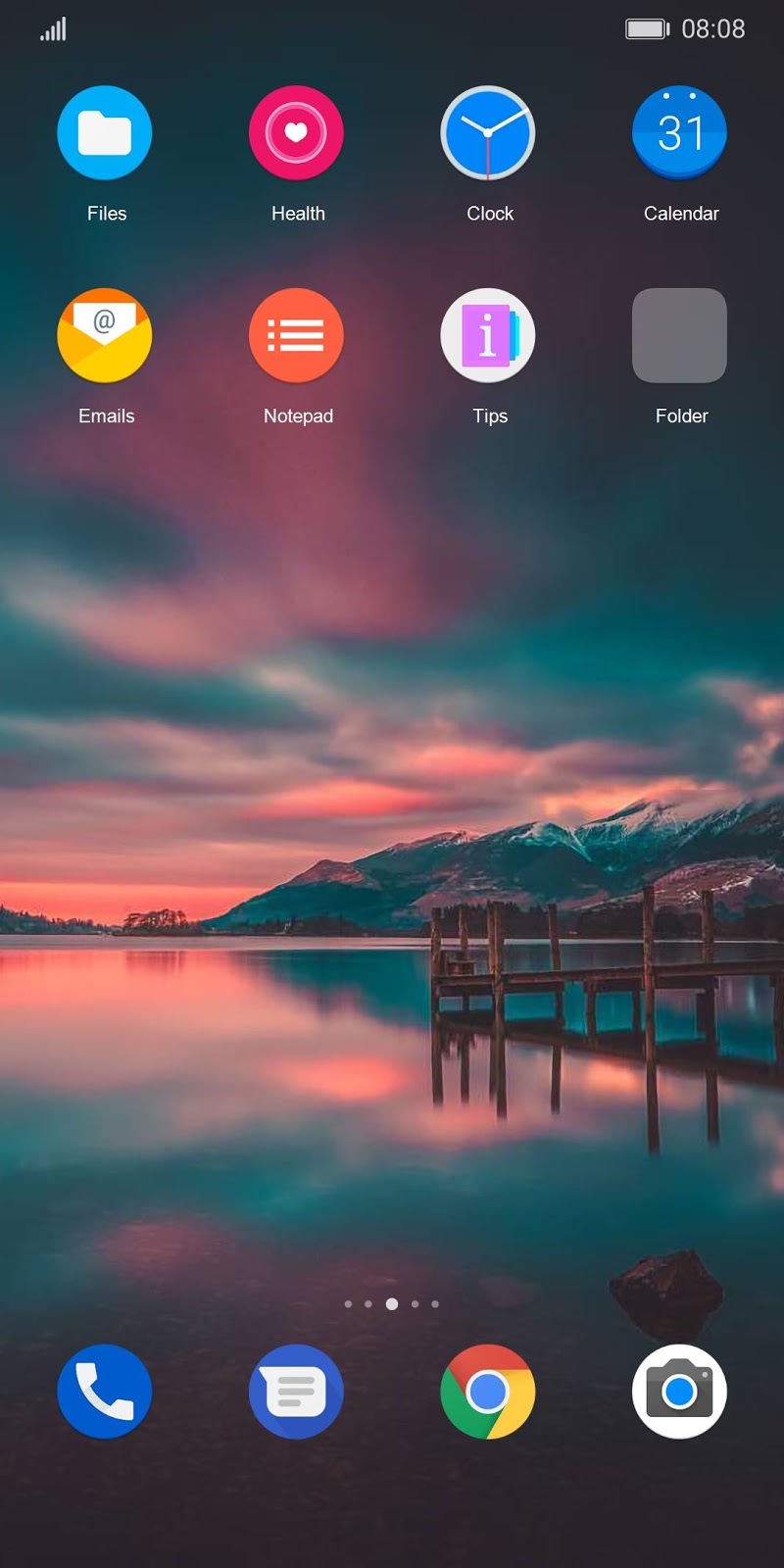The image captures a screenshot of a mobile phone's main screen set against a scenic background of a Norwegian lake. The serene landscape features a dock extending into the still waters, an orange glow blanketing the scene, with a cloudy sky and mountainous terrain adding depth to the picturesque view.

At the top left corner of the phone screen, a service bar is displayed with all five bars full, indicating a strong signal. On the top right, the battery icon shows it's fully charged, and the time is shown as 8:08.

The layout comprises two rows of app icons situated just below the status bar. The first row includes:
- A blue circle with a file icon labeled "Files."
- A pink circle with a white heart icon labeled "Health."
- A blue clock icon labeled "Clock."
- A blue circle with the number 31, indicating the "Calendar."

The second row contains:
- A yellow box featuring a piece of paper with the letters "Ad," labeled "Emails."
- An orange box with three bullet-pointed lines, labeled "Notepad."
- A white box with a pink square inside containing the letter "I," labeled "Tips."
- A gray box simply labeled "Folder."

At the bottom of the screen, four icons are aligned horizontally:
- A phone icon in the bottom left corner.
- A messenger icon with a blue background next to it.
- A Google Chrome icon positioned centrally.
- A camera icon with a white background, black camera, and blue lens.

This organized setup, coupled with the tranquil background, offers a harmonious blend of technological convenience and natural beauty.